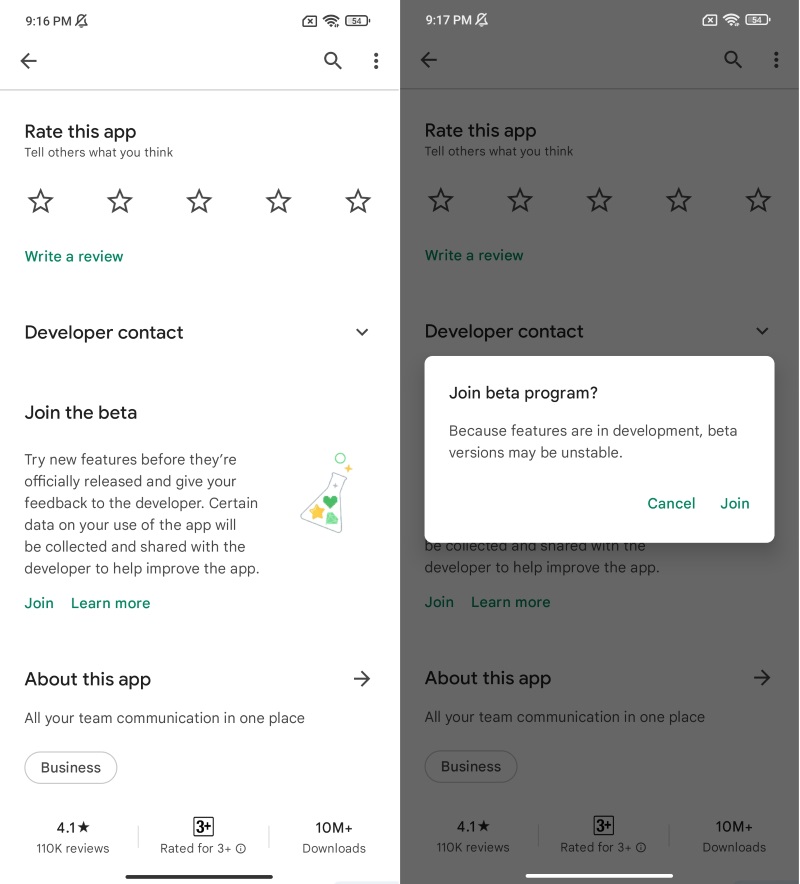The image shows two screenshots from an Android phone displaying the Google Play Store. The screenshots are positioned side-by-side for comparison. 

The left screenshot showcases the app's main rating and review section. It prompts users to "Rate this app" and "Tell others what you think." Users can select a star rating and write a review. Below this section is an expanded "Developer contact" option, featuring a "Join the beta" invitation. This option encourages users to try new features before their official release and provide feedback to the developer. It notes that data on app usage will be collected and shared with the developer to aid in improving the app. Users have the options to "Join" the beta or "Learn more." An "About the app" section details that the app has a rating of 4.1 out of 5 stars based on 110,000 reviews, is suitable for ages 3 and up, and has over 10 million downloads.

The right screenshot displays the result of clicking the "Join beta" button. A dialogue box asks, "Join beta program?" emphasizing that beta versions may be unstable as features are in development. Users must click "Join" to proceed. The background of this screenshot is dimmed with the dialogue box in the foreground standing out in bright white. Both pages feature a mostly white background with black text, accented by teal elements. The overall theme suggests that joining the beta can provide access to new features, albeit with potential instability.